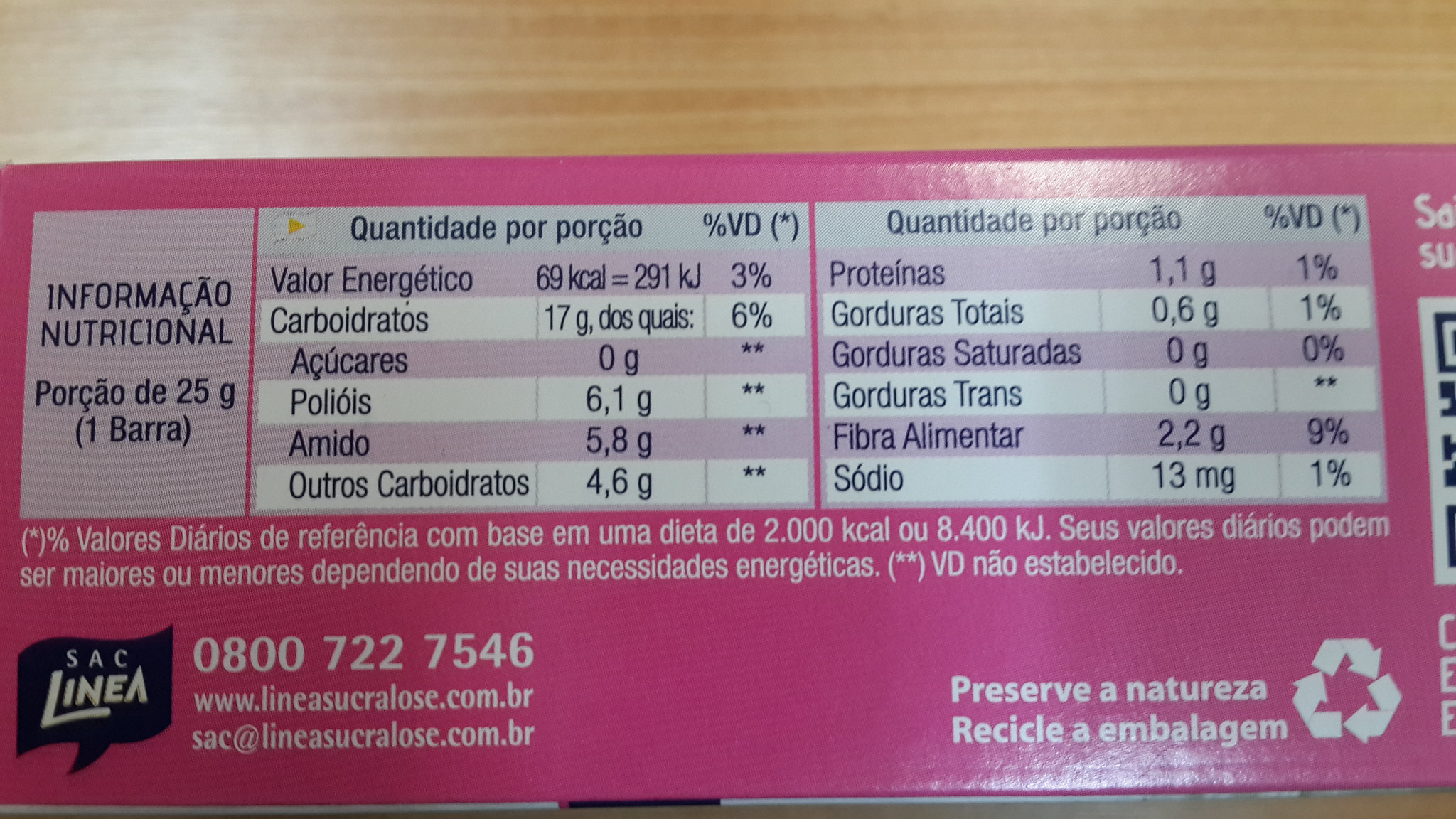In this image, we see the back of a pink package, likely a product manufactured by the company Sac Linea, whose logo is displayed prominently in the bottom left-hand corner. The text on the package is primarily in Spanish. The "Nutrition Facts" section stands out in black letters, labeled as "Información Nutricional." The bottom right-hand corner features a recycling symbol, indicating the package's recyclability. Additionally, a contact phone number, 0800-722-7546, is printed on the package, accompanied by several website URLs below it. The package itself rests on a light brown table, providing a neutral background that contrasts with the vibrant pink color of the package.